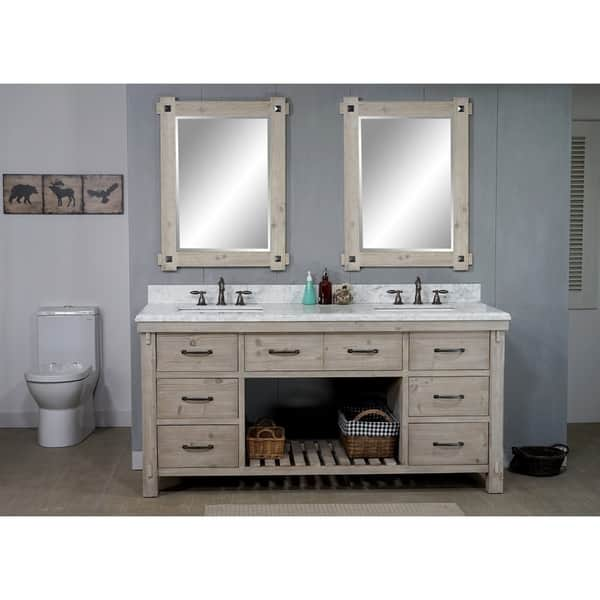This detailed photograph showcases a spacious, modern bathroom with a clear emphasis on the stylish double-sink vanity area. The vanity features a white marble countertop with sleek metal faucets and handles, and is equipped with a total of seven drawers, adorned with dull brass handles for a classic touch. The vanity is constructed from light taupe or whitewashed wood, and beneath it lies a recessed area housing two wicker baskets, one plain and the other lined with blue and white cloth. Centrally positioned on the counter are three soap bottles, flanked by two rectangular wooden-framed mirrors that mirror the vanity's finish. The bathroom walls are predominantly gray, contrasting with the lighter lilac hue on the adjacent walls. On the left side of the image is a modern, white porcelain toilet adjacent to an artistic piece featuring black silhouettes of a bear, a moose, and a flying eagle, enhancing the rustic aesthetic. The wooden floor adds warmth to the space, balancing the cooler tones of the paint and tile flooring. This meticulously designed bathroom could easily feature in a high-end catalogue for bathroom fixtures or home decor, offering both functionality and style.